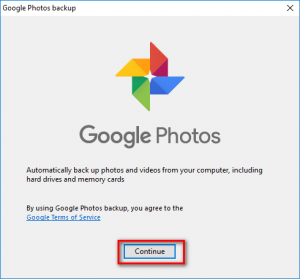This image is a screenshot of a pop-up on a computer screen. The pop-up features a white header with the text "Google Photos Backup" in black on the left side, and a gray 'X' button on the right side for closing the notification. The body of the pop-up has a light gray background. Centered at the top is a multicolored logo composed of several triangles arranged in a radial pattern, forming a subtle four-pointed star shape in the center where the light gray background shows through. The triangles are colored orange, red, blue, and green, arranged clockwise starting from the top-left.

Below the logo, large gray text states "Google Photos," with "Google" in bold and "Photos" in a regular font. Underneath this, there is smaller black text in two lines that reads: "Automatically back up photos and videos from your computer, including hard drives and memory cards." Further below, there is more black text stating, "By using Google Photos Backup, you agree to the," followed by a blue, underlined text "Google Terms of Service."

At the bottom center of the pop-up, there is a gray button outlined with a thin blue line and containing black text that says "Continue." This button is further accentuated by a thin red rectangle around it. The entire pop-up is bordered by a very thin blue line.